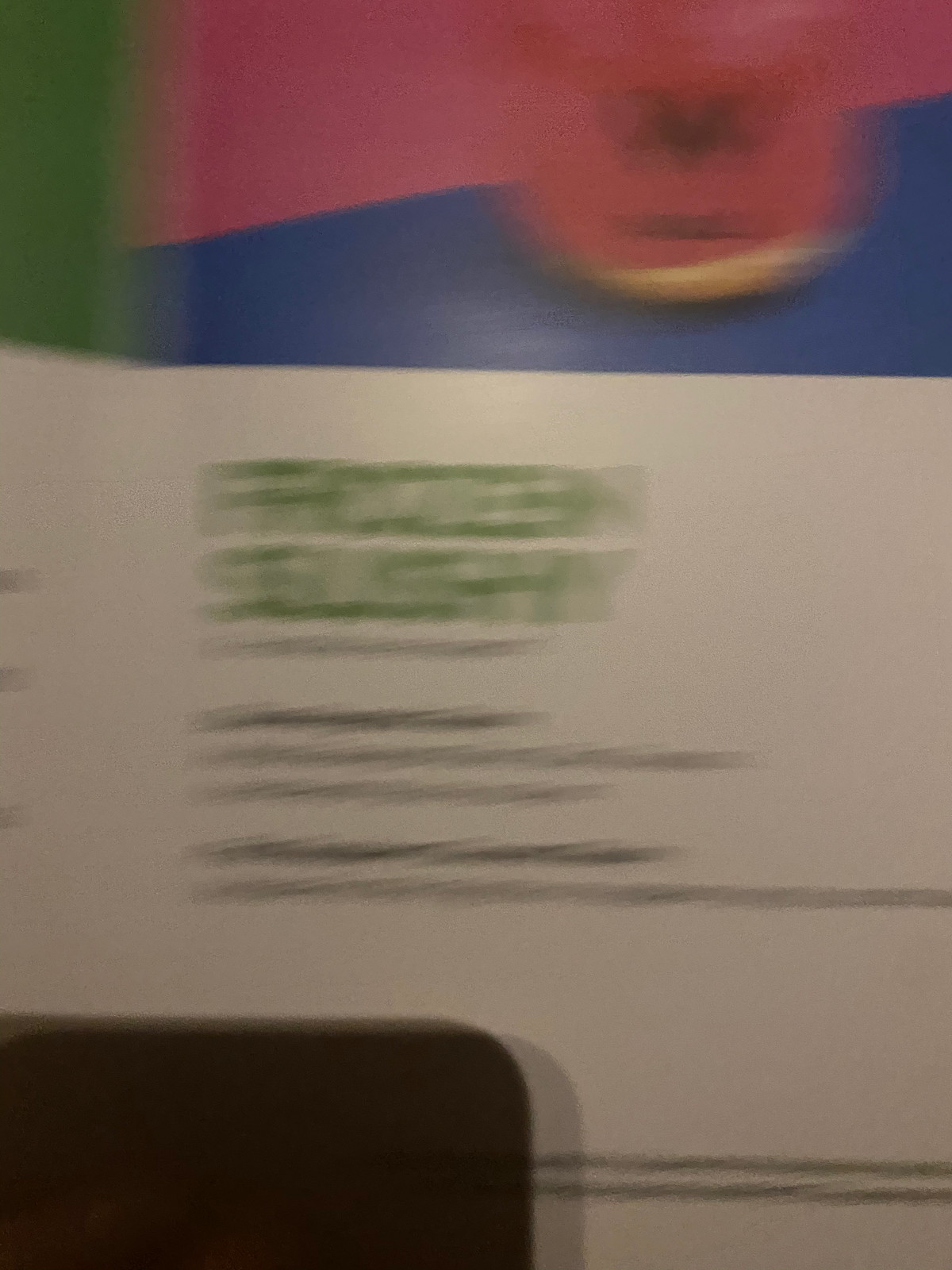This photograph showcases a somewhat blurry and grainy image of packaging. At the top left, there is a lime green box, followed by a pink section, with a blue strip below it. Within the center of the blue strip, there is a pink circle that displays black text, and at the bottom of this circle, there is a touch of tan. The lower part of the image predominantly features a white background. At the very top, large green text is visible, followed by very blurry black text underneath. Centrally positioned and resting on the packaging is a brown, square-shaped object which casts a shadow onto the white surface below. Additionally, a small area of light is visible reflecting off the white background.